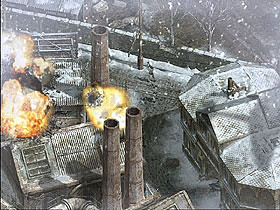An animated graphic presumably originating from a video game depicts a scene characterized by a pervasive grayish tint. The focal point of the image is a warehouse-like building situated on a snowy rooftop. This structure features two prominent smokestacks arising from its rooftop towards the bottom center of the image, with an additional smokestack visible. Three vibrant fireballs, colored in hues of yellow and orange, create a striking contrast as they appear to the middle left of the frame.

Adjacent to the warehouse, a small house can be seen positioned directly in front and to the right. Another house is partially visible behind the smokestacks on the left side. Trees are scattered throughout the scene, adding a touch of natural element to the industrial setting. The image is further brought to life by a gentle snowfall, creating a serene wintery atmosphere. In the foreground, a couple of diminutive human figures are discernible, adding scale and a hint of activity to the intricate landscape.